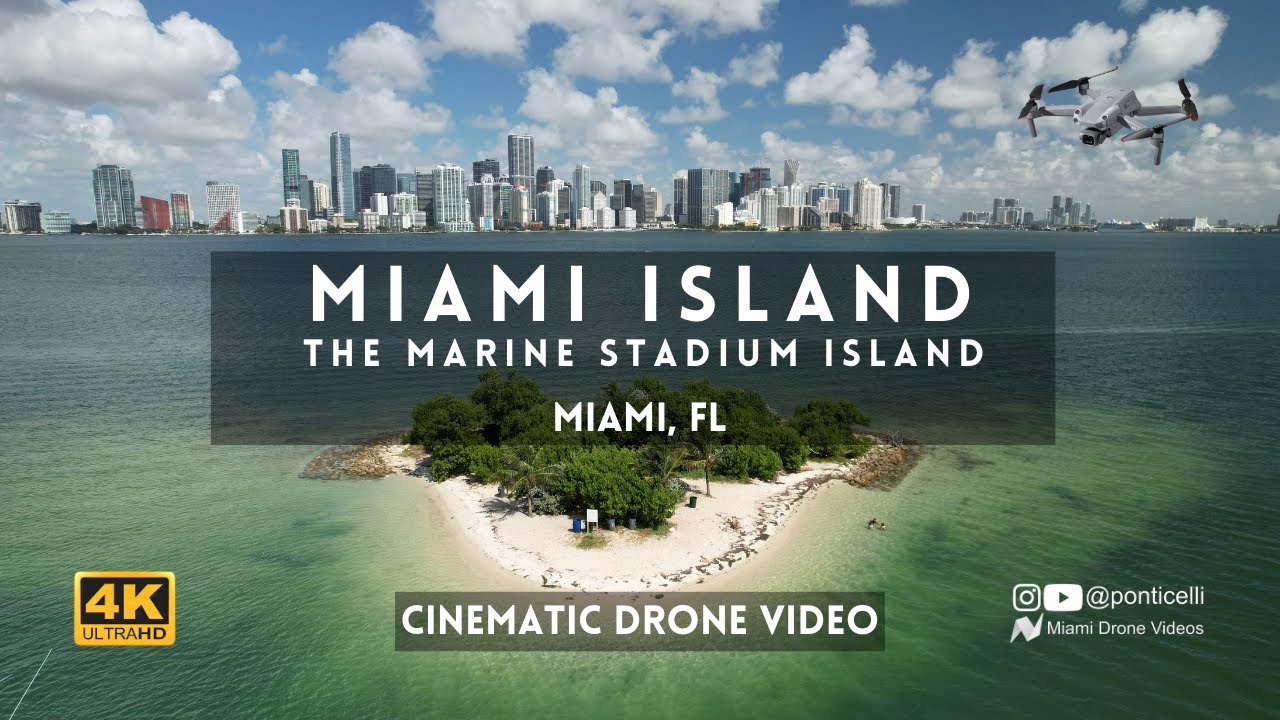The image depicts a promotional poster for "Miami Island," specifically "The Marine Stadium Island" in Miami, Florida. The photograph, which seems computer-generated, shows a small, triangular island with sandy beaches and green trees, set against the transparent waters of the ocean. In the foreground, there is bold white text centered in a translucent black bar stating "Miami Island, The Marine Stadium Island, Miami, Florida," with "Cinematic Drone Video" written below. The left side features a 4K Ultra HD logo in gold and black lettering, while the right showcases Instagram and YouTube logos with the handle @Ponticelli and the caption "Miami Drone Videos." The background reveals the city of Miami, characterized by many skyscrapers, under a blue sky filled with fluffy white clouds. A white drone is visible flying in the top right corner.